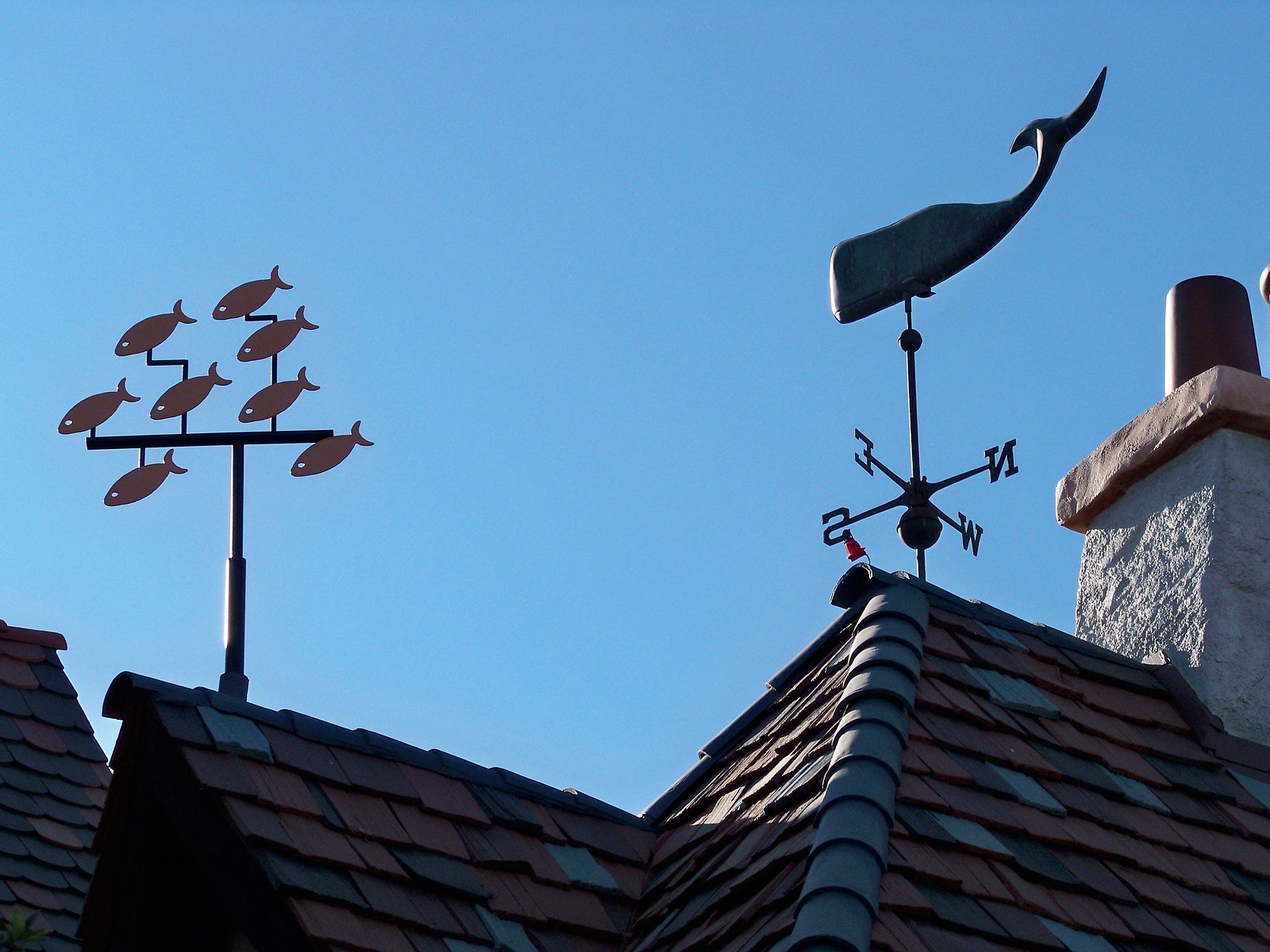The photograph, a color image shot in landscape orientation with the camera angled upwards at a 45-degree tilt, captures a detailed view of a multi-peaked rooftop against a clear, cloudless blue sky. The roof is clad in overlapping shingles of teal and dark reddish-brown hues. Dominating the right side of the frame, although partially cut off, is an off-white chimney. This chimney features a light pinkish band around its top and is capped with a dark brown cylindrical flue. Beside this chimney, perched on the rightward roof pitch, stands a weather vane topped with the silhouette of a whale, its tail playfully flicked upwards to the sky. On the left side of the roof, near the edge of the frame, another weather vane features a school of eight metal fish, arranged in a coordinated pattern with pointed struts, each fish angled slightly downwards. The striking, uninterrupted expanse of blue sky provides a serene backdrop, emphasizing the intricate elements and vivid colors of the rooftop details.